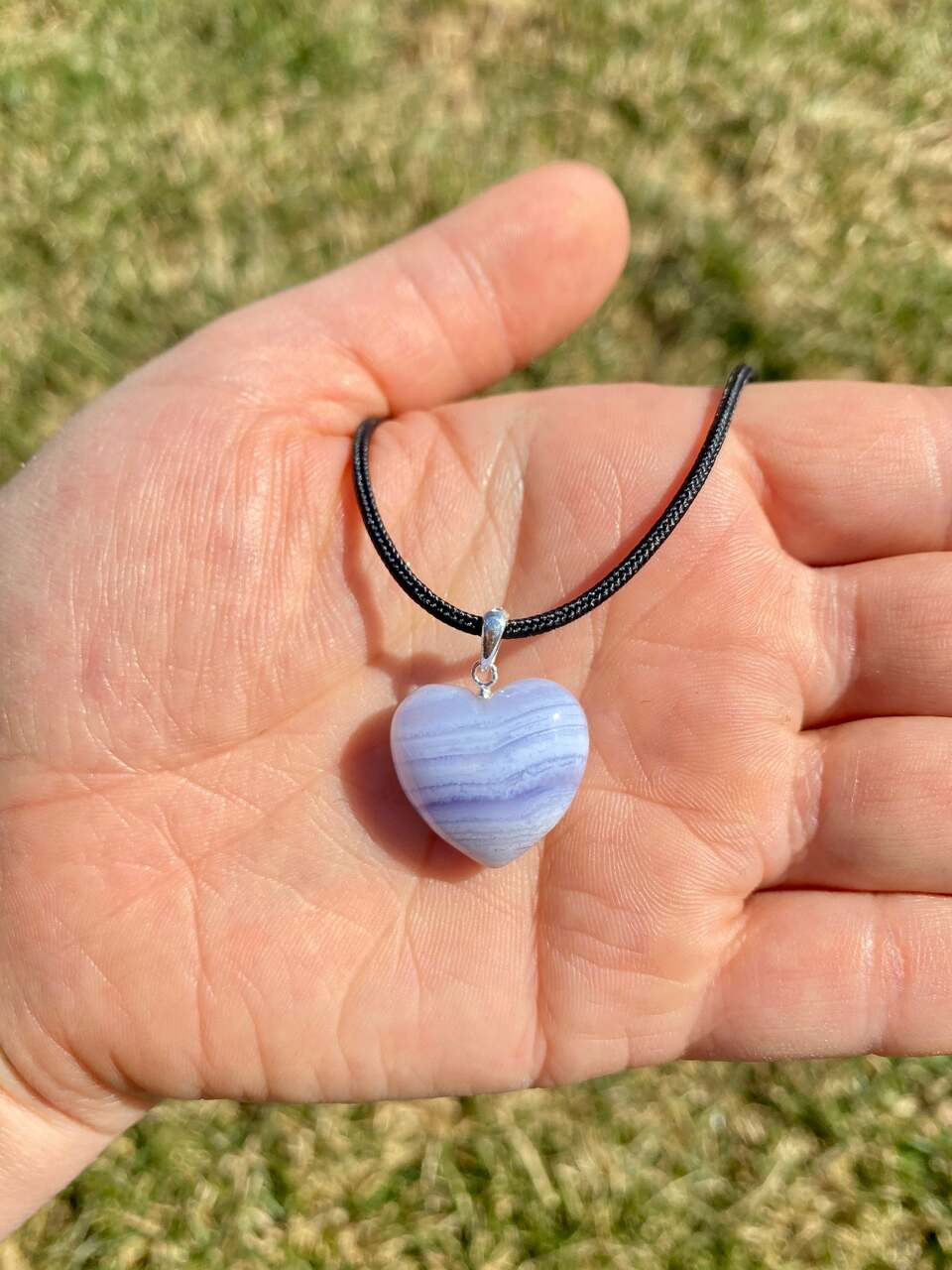This image captures the close-up of a left hand with a black braided cord necklace delicately held between the thumb and palm. The hand's skin is fair and detailed with visible wrinkles and lines. The necklace features a heart-shaped pendant, which is the focal point of the photo. The pendant is an exquisite piece with horizontal stripes in varying shades of purple, ranging from lavender to a deeper purple, interspersed with hints of blue. The heart pendant has a textured, almost stone-like appearance, possibly amethyst, and is secured to the black cord with a small silver hook and loop. The background, slightly out of focus, reveals a grassy field with patches of green and sunburned yellow, suggesting a sunny day. The pendant, resting in the center of the open palm, shines with its vibrant hues against the natural backdrop.